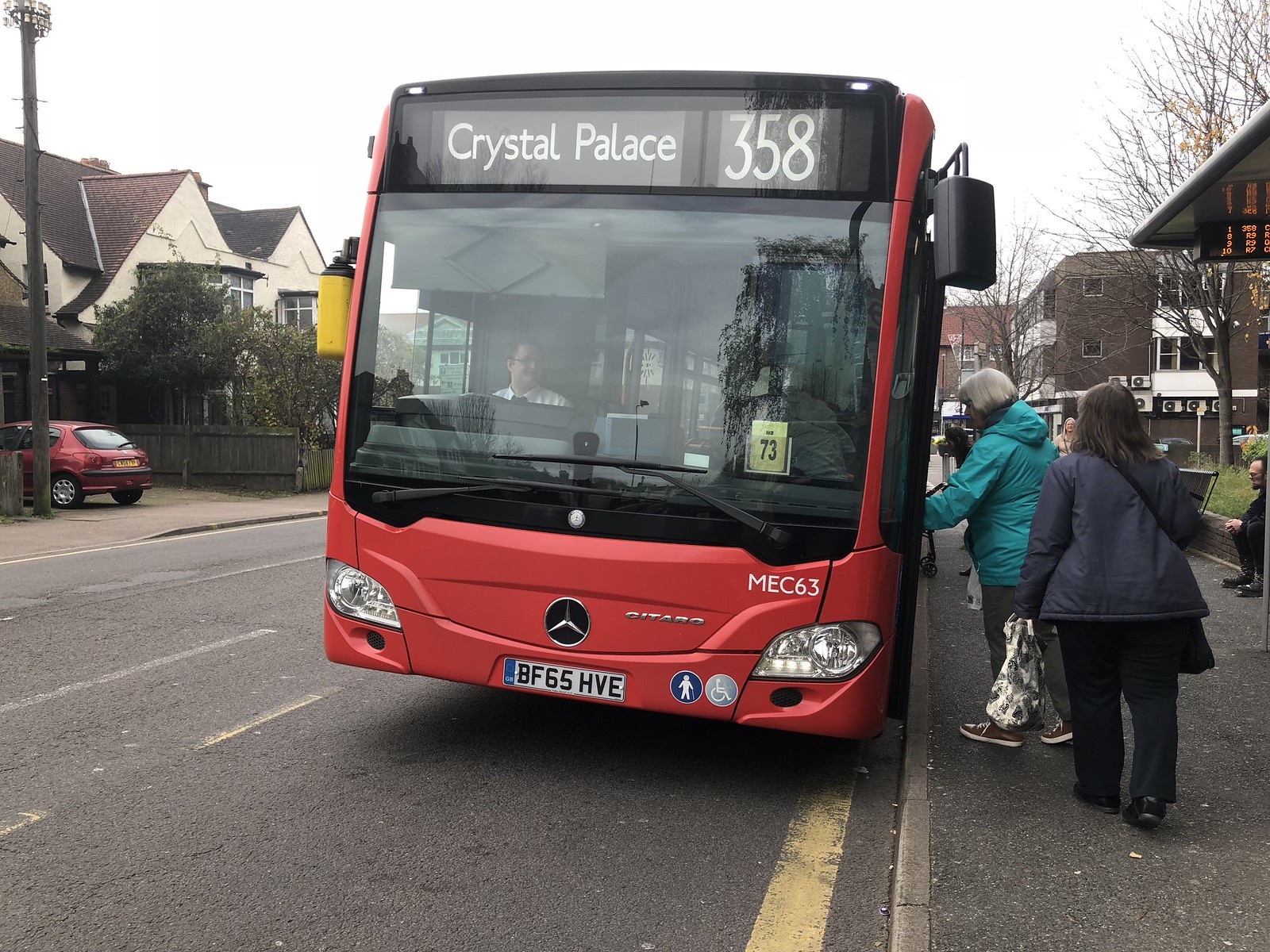In this detailed image description, we see a red, single-decker City Transit bus in a residential neighborhood, identifiable by the houses, parked cars, and an apartment complex visible in the background. The bus, manufactured by Mercedes, prominently displays the Mercedes emblem just above its white license plate reading BF65 HVE. The route number on the bus is 358, and the destination is Crystal Palace, as indicated by the text on the front. The bus also features the text "MEC63 Sitaro" near the entry door on the front right corner.

The bus driver, seated on the right side, aligns with the English setting suggested by the English license plate. Two women are boarding the bus from the right side; the woman in the front has white hair and is donned in a bright turquoise rain jacket, while the woman behind her wears a dark blue rain jacket, carrying a black purse and several grocery bags. The image captures a cloudy day, with the same asphalt used for both the sidewalk and the street. Although there are other people in the background, their details are obscured.